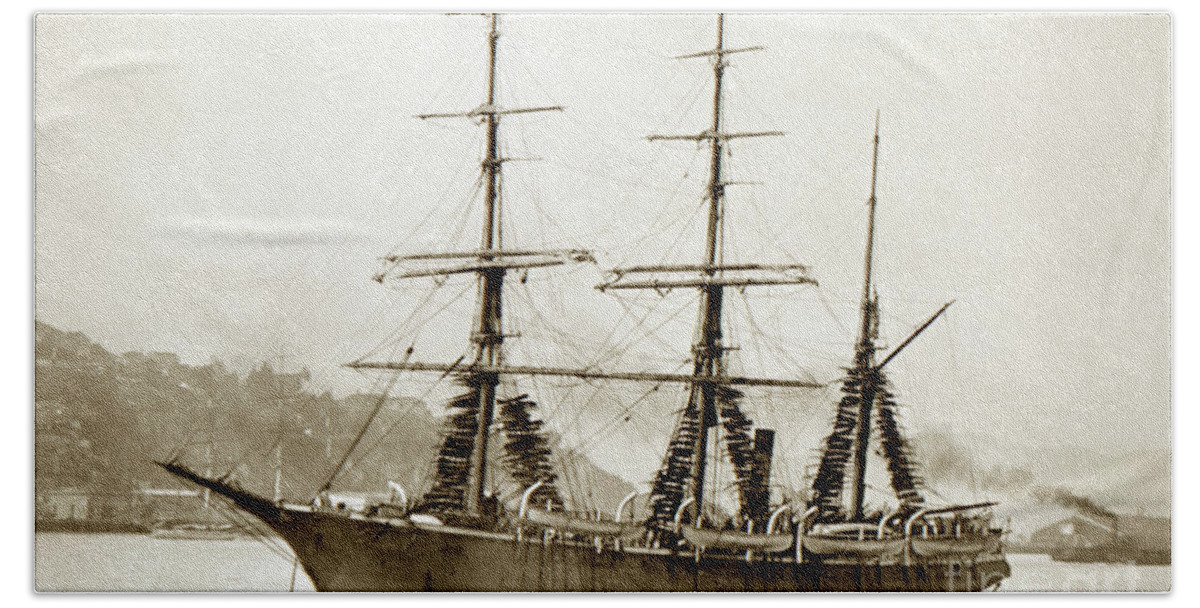This detailed black-and-white photograph depicts an old, sepia-toned wooden sailing vessel, centrally framed and situated in calm waters. The ship, which could date back to the late 1800s or early 1900s, is notable for its three large masts devoid of sails but adorned with a network of ropes and cables. It appears aged and possibly deteriorated, evoking images of a pirate ship. Four smaller canoe-like lifeboats hang on the left side of the hull. The background reveals a misty, partly obscured coastal village nestled within a mountainous landscape. In this foggy setting, the outlines of buildings and houses on the hills are visible but blurry. Faintly, a tugboat emits black smoke from its stack, contributing to the weathered, historical ambiance. The sky appears clear but grey, typical of old photography. There are hints of human presence on the ship, although the individuals are too faint to discern clearly due to the photograph's age and style.